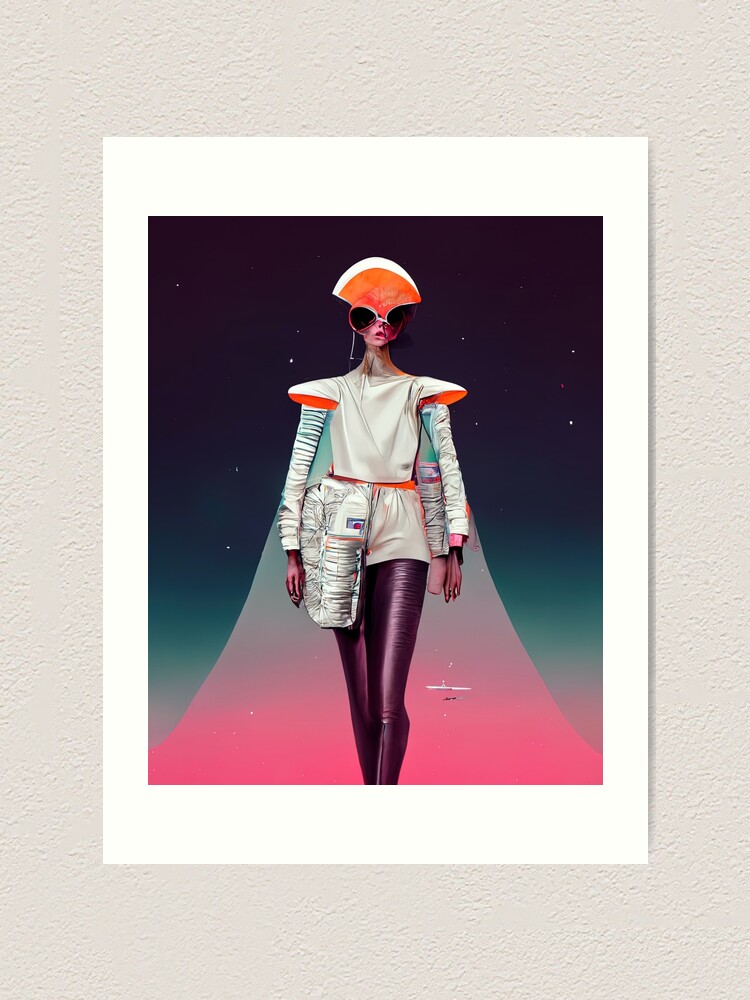The image appears to be a digitally created photograph of a model walking on a runway in a futuristic outfit. The model, depicted in the center, is dressed in purple-black pants that extend to the ankle, paired with a white onesie-type outfit featuring high-cut shorts and prominent shoulder pads. The outfit is further detailed with tight-fitting, light white sleeves, and the model's face is mostly concealed by an orange and white semi-round hat or face mask, enhancing an alien-like appearance. The model's slender figure and straight posture, with hands at their sides, contribute to the otherworldly aesthetic.

The background is a striking combination of colors: a pink runway leading into a gradient of turquoise that transitions into a starry black sky. There is a white border framing the image, surrounded by a cream-textured outer border that resembles cardboard. This layered presentation gives the overall appearance of being within a stylized picture frame. The vivid hues and the surreal design elements affirm the image's AI-generated, animation-like quality, crafting a scene that is both futuristic and slightly surreal.